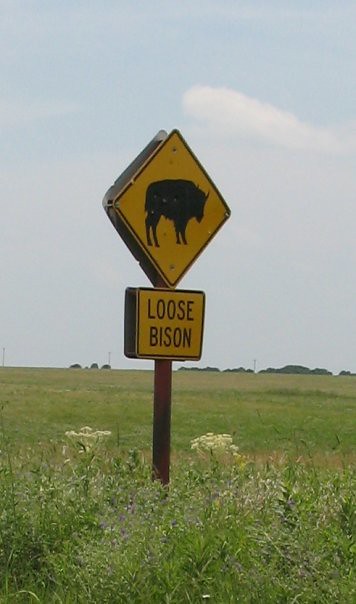This image captures a verdant field extending into the horizon, with clusters of trees and bushes dotting the distant landscape. The lush green expanse is prominently featured in the foreground, bustling with a variety of grasses and white umbelliferous plants, adding texture and diversity to the vegetation. Dominating the middle ground is a brown wooden post supporting a dual-sided notice. The notice is composed of two parts: the upper section is a diamond-shaped sign standing on its point, vividly displaying a black silhouette of a bison against a bright yellow background. Below the diamond, a rectangular sign clearly warns in bold letters, "Loose Bison." Intriguingly, despite the notice's apparent need for visibility, it is situated not by a roadside but rather in the midst of the open field, heightening the sense of caution and curiosity.